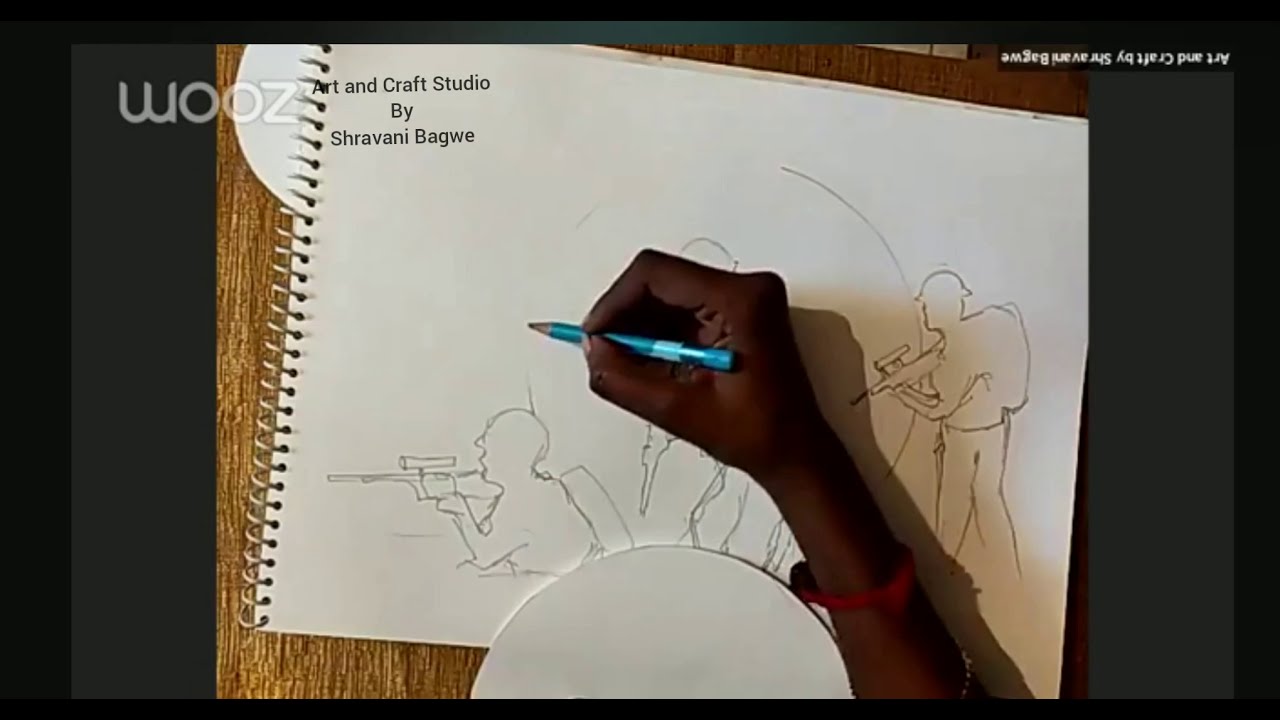The photograph captures a close-up of a dark-skinned hand, adorned with a red bracelet, holding a blue pencil with possible accessories at the back. The person is meticulously sketching on a white piece of paper within a sketchpad bound by binder rings. The sketchpad rests on a medium-brown wooden table. The artwork in progress depicts military figures; there are outlines of soldiers and snipers equipped with rifles, with three figures already visible and a circle being carefully added. At the top of the sketchpad, black text reads "Art and Craft Studio by Shravani Bagwe," while the upper left corner features a semi-transparent white logo with the text “WOOZ.”